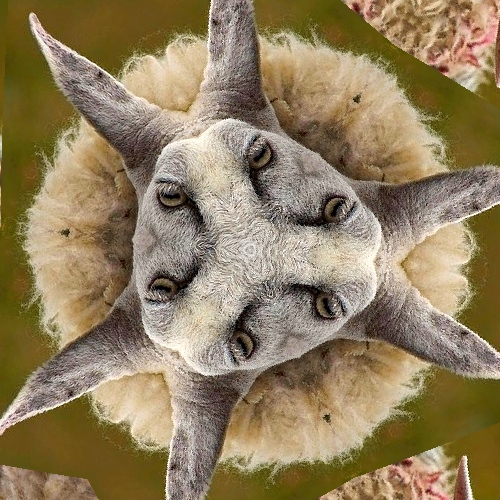The image features a kaleidoscopic composition of three animal faces arranged in a triangular formation, converging at a shared central point where their noses would be. The animals have light gray faces with darker gray ears that form a distinctive Y-shape. Their eyes are oriented towards the center, giving the illusion of a single face made from multiple creatures. The background is a vivid mix of lime green with subtle pink and brown hues, resembling a textured sheep's wool or fur. The entire arrangement has a star-like or circular pattern, producing a mesmerizing, almost surreal visual effect. Additional elements include hints of feathers and possibly floral designs, adding complexity to the olive green and yellow-tinted backdrop. The image combines rabbit-like ears, eyes reminiscent of various animals, and intricate fur details to create a unique, detailed piece of art.